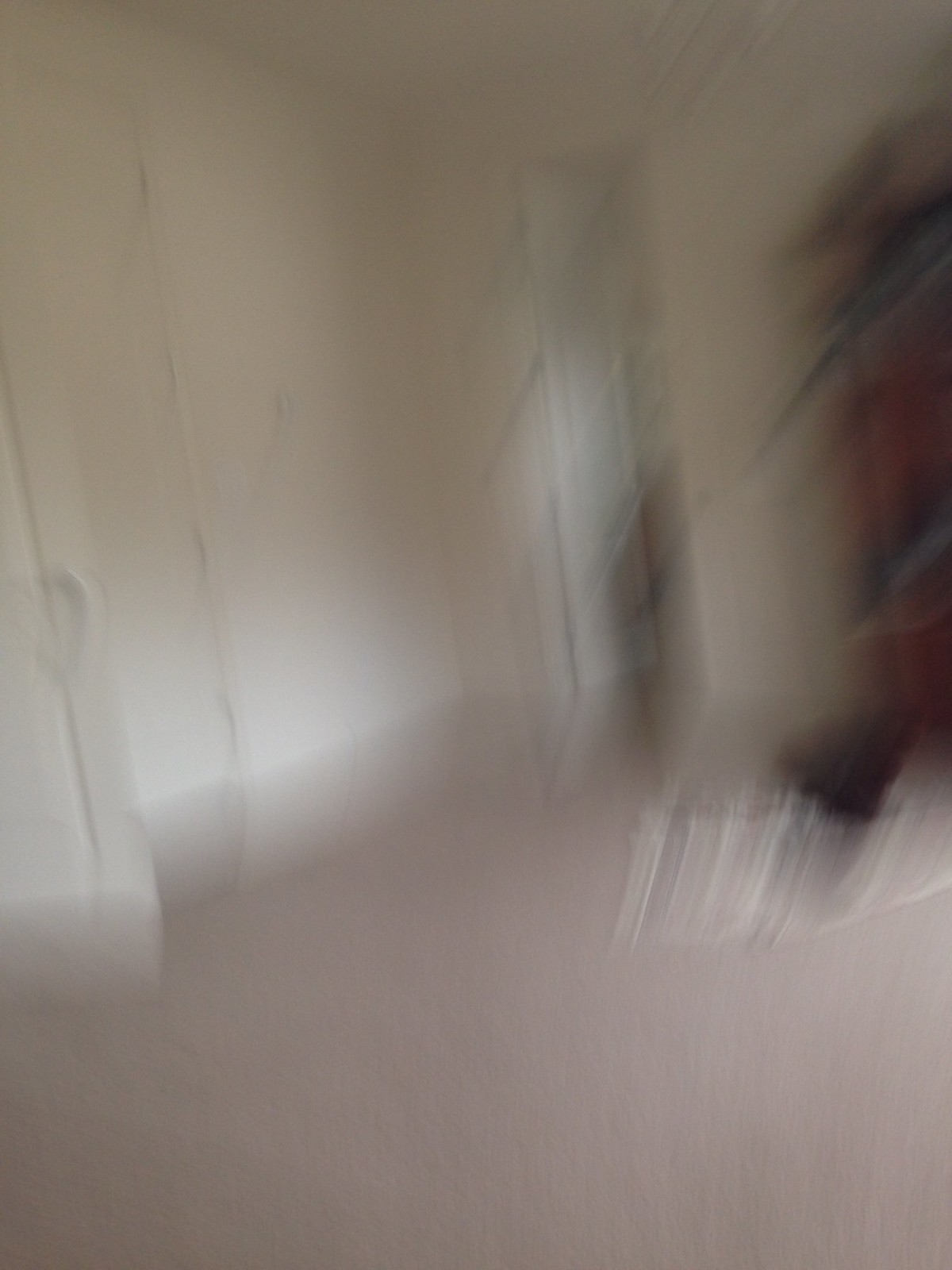A highly indistinct, blurry color photograph depicts an indoor room with white walls. At the back of the image, an open doorway is faintly visible. The flooring also appears to be white. On the far right side of the photograph, there is an ambiguous shape with black and red hues, though the extreme blurriness makes it difficult to ascertain its identity. The image contains no text, people, plants, animals, buildings, signs, flags, or banners.